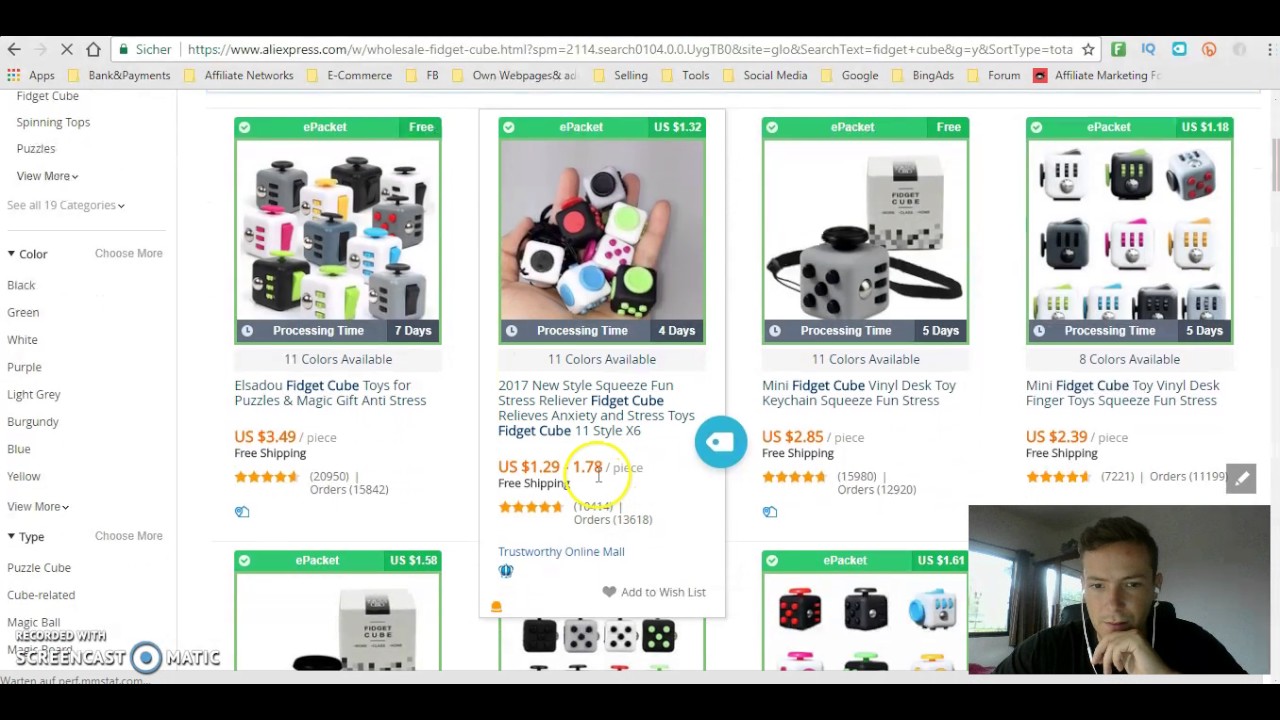This image showcases a screenshot of the AliExpress website, specifically on a page dedicated to wholesale fidget cubes. At the top of the browser window, the address bar indicates the URL: aliexpress.com/wholesale-fidget-cube. The main section of the screenshot displays various images and search results for fidget cubes. Of particular interest is the bottom right corner, where a gentleman appears to be speaking or describing the products visible on the screen. 

On the left side of the page, there is a comprehensive filtering menu allowing users to refine their search by categories such as spinning traps and puzzles, with a total of 19 categories available. Additionally, users can select their preferred color and type of fidget cube, with options including puzzle cubes, cube-related items, and magic balls. Among these selections, four options are fully visible, while three more are partially displayed below them. Highlighted in the results is the "2017 New Style Squeeze," suggesting a focus on describing or promoting this particular item.